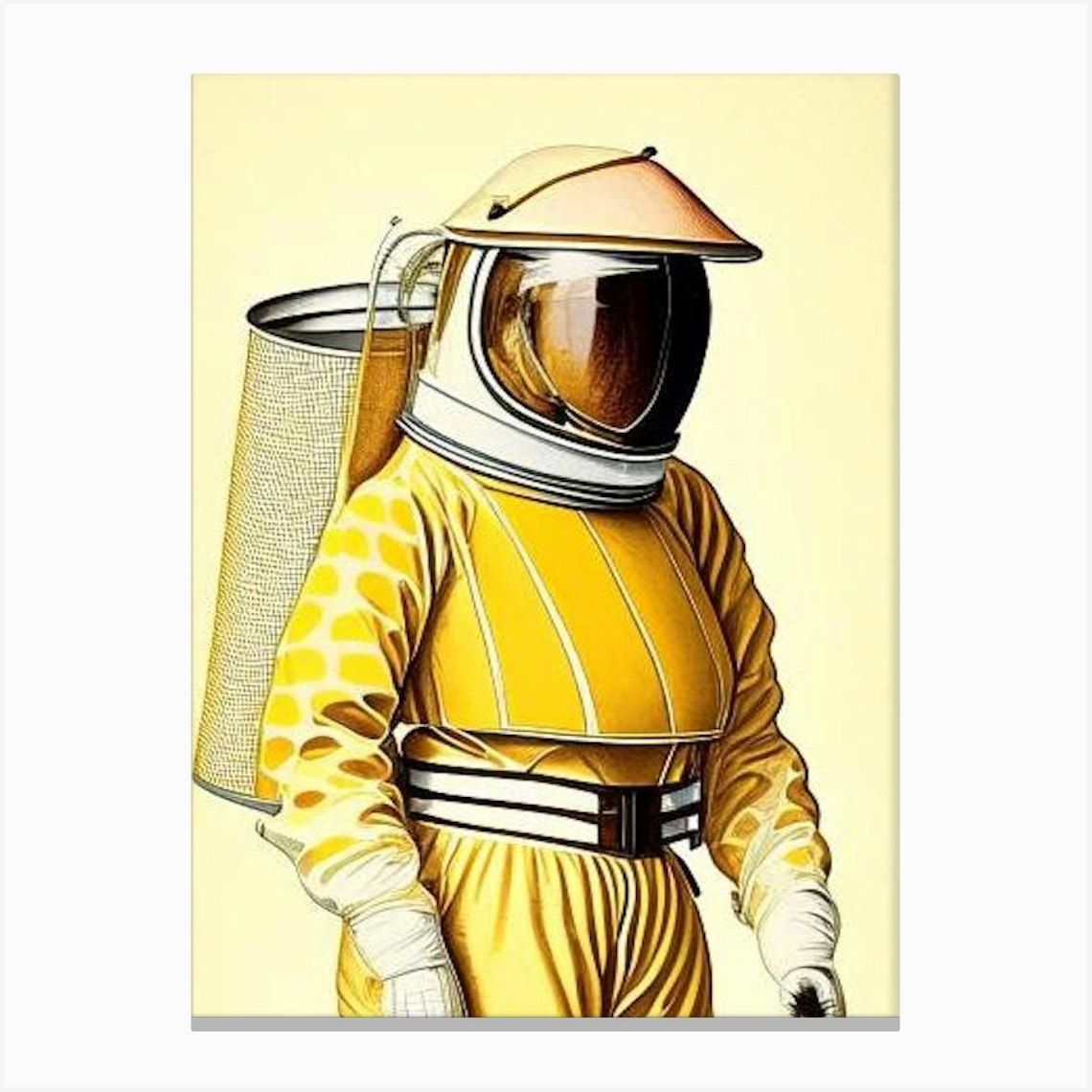This is a detailed illustration of a futuristic, bee-like figure, known as a V-keeper, dressed in a vibrant, golden-yellow beekeeping suit set against a vivid yellow background that resembles a vintage canvas print. The V-keeper's suit features a honeycomb pattern comprising of large, orangish-yellow circles and blots separated by beige lines on the arms. His torso is protected by a dark yellowish-gold plate adorned with white stripes. The ensemble includes a wide black and white belt with a prominent black clasp, and the trousers are a matching yellow. His hands are sheathed in thick white gloves. 

On his back, he carries a long cylindrical container, sprayed with a light, almost-opaque yellow and dotted with black. This container, likely used to distribute calming smoke over beehives, is held in place by an intricate apparatus that includes a silver bar lined with dark yellow, almost gold fabric. His headgear is reminiscent of a space or diver's suit with a light brown hat, a white protective covering, and a glass visor transitioning from black to dark brown, reflecting sunlight at its edge. This highly detailed depiction combines elements of vintage art with a futuristic twist, giving the V-keeper an otherworldly yet distinctly beekeeping appearance.